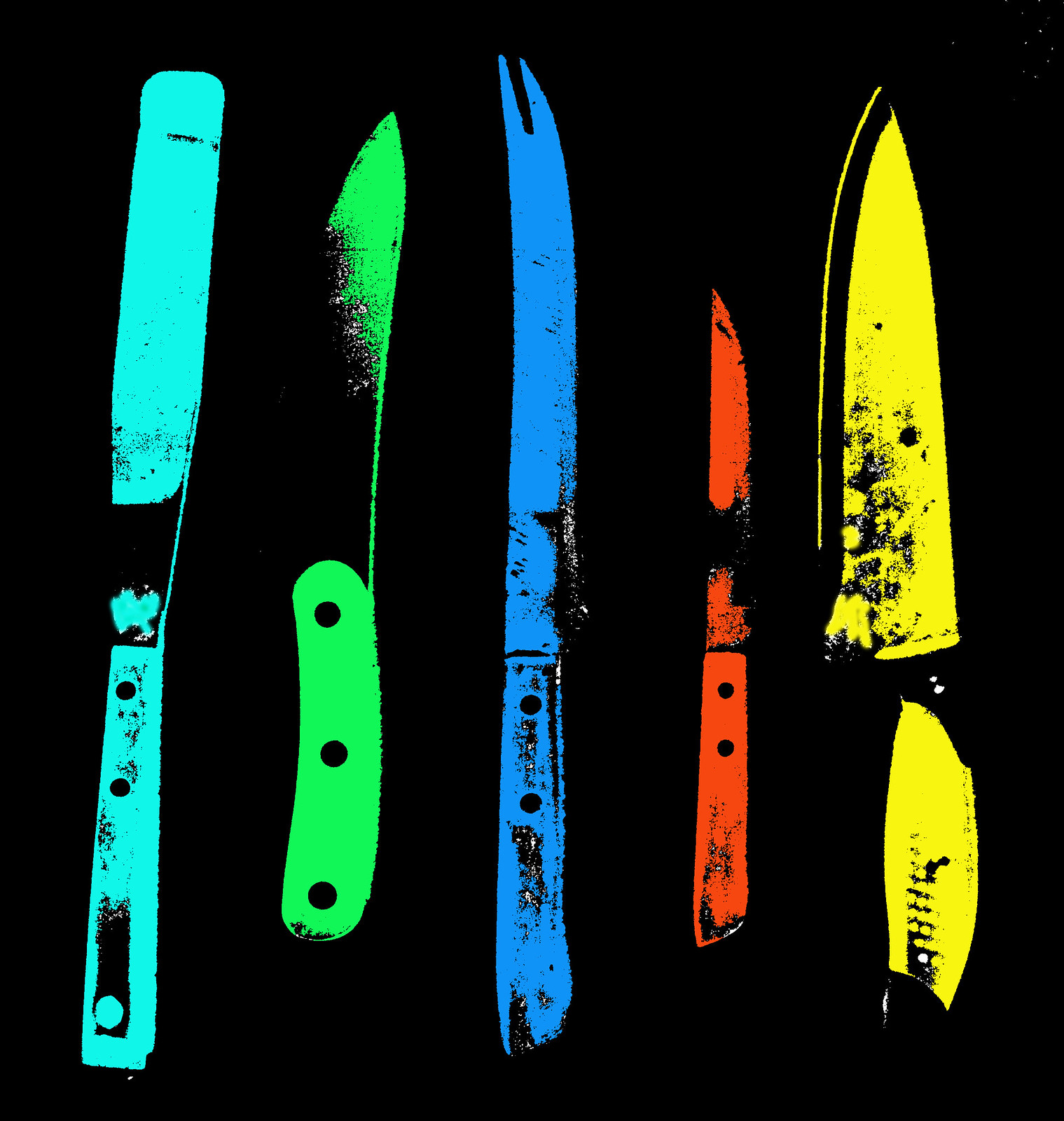This intricate image resembles a piece of vivid pop art, featuring five distinct kitchen utensils splayed vertically against an all-black background. The colors are vibrant and neon-like, giving an artistic, almost spray-painted effect. On the far left, a turquoise blue utensil stands out, resembling a spatula or butter knife with a handle and a blade akin to a cake scraper. Next to it, a neon green knife with a slightly curved handle, adorned with three black dots, merges partially with the black background, except for its sharp green tip. The middle utensil is a long, blue carving knife, distinguished by two prongs at the tip. Adjacent to it, a bright red knife, likely a serrated steak knife, draws attention. Finally, on the far right, a large yellow chef's knife completes the tableau. The knives' partial outlines and high-contrast colors against the pitch-black backdrop create a striking, almost silkscreen print effect, reminiscent of Andy Warhol’s iconic style.